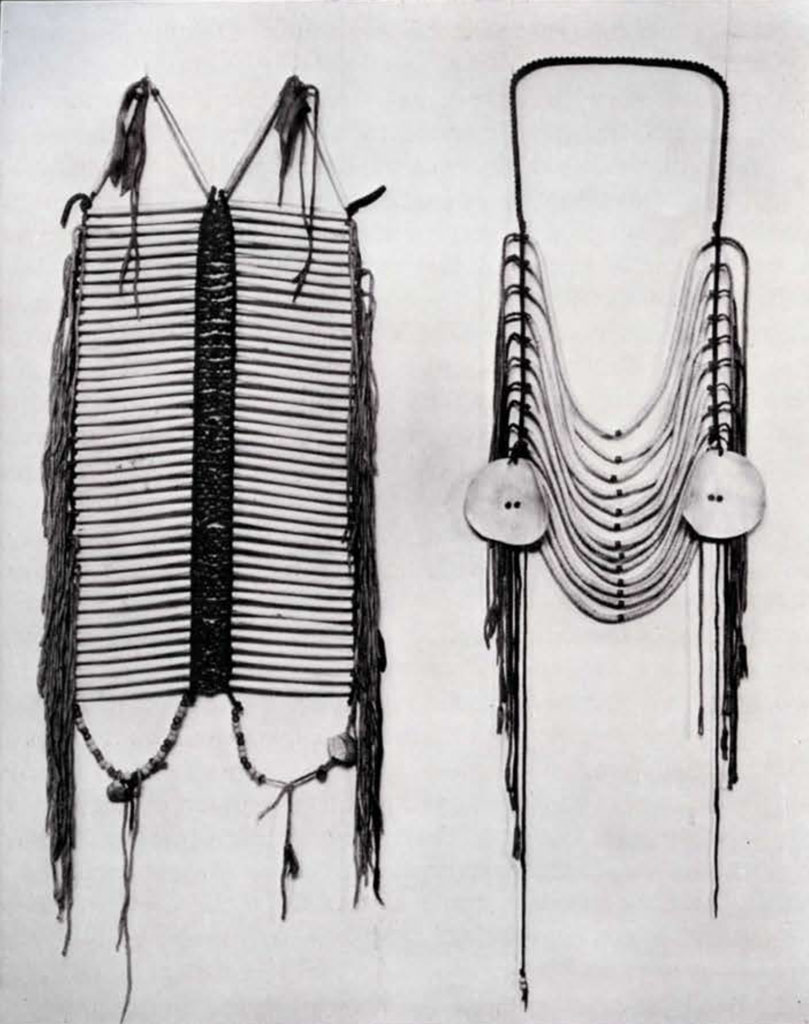This photograph captures two distinct Native American-inspired wall hangings against a white backdrop, suggesting they might be traditional decorative pieces or ceremonial items, possibly resembling breastplates. The left wall hanging, mounted on two nails, features two upward-pointing triangular sections at the top, transitioning into horizontal rows of small wooden pieces that mimic the arrangement of an old washboard or chest guard. It boasts black knots running down the center and is flanked by black-trimmed ropes that end in hanging beads. The material extending from the sides resembles hair, adding texture and complexity to the piece.

In contrast, the right hanging, also secured by two nails, is characterized by its simpler design. It consists of a central long rope with numerous strings radiating downward, highlighted by two large white circles resembling the cut centers of apples or oversized earrings. These elements punctuate the otherwise minimalist fringe that cascades to the bottom, creating a visually engaging display alongside its more intricate counterpart.